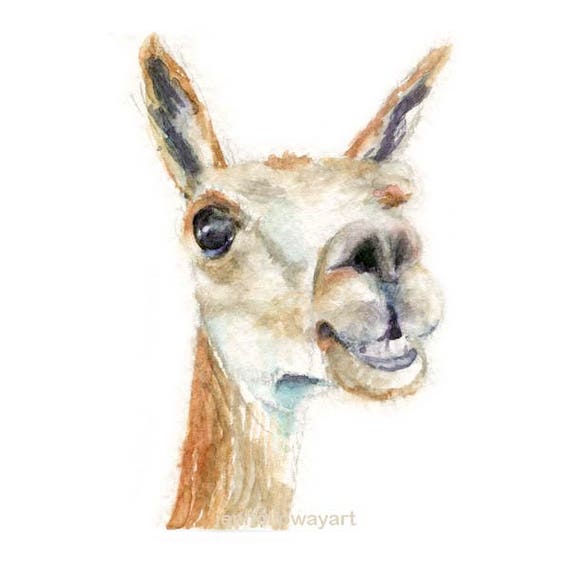This image is a detailed watercolor-style illustration featuring the face and partial neck of an animal, prominently labeled with a "Wayart" logo. The animal has characteristics that blend traits of a donkey, camel, and llama. It has one visible big brown eye, a slightly open mouth showcasing a black bottom lip and white teeth, and both ears are prominently displayed with a mix of black, brown, tan, and dark gray colors. The face is primarily white with hints of tan and brown speckles, while the neck is a mixture of tan, cream, white, and grayish-blue/teal, which may represent shadows. The animal’s expression is cheerful and happy, with a smile that adds to its friendly demeanor. The background is white, complementing the watercolor texture and strokes that give depth to the illustration.